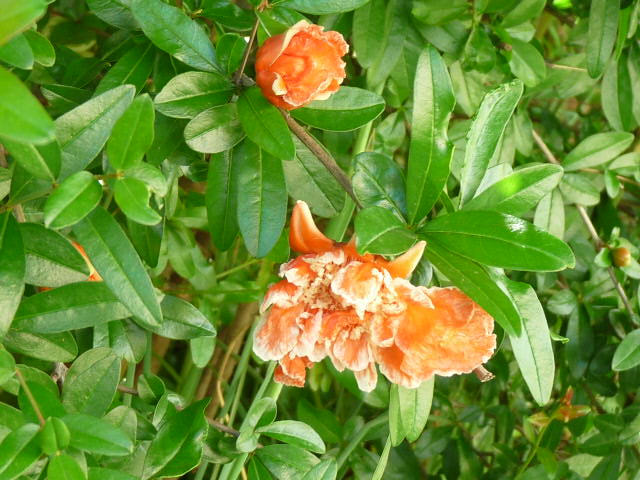This vivid daytime photograph captures an outdoor setting dominated by lush greenery and vibrant colors. Central to the image is an orange flower, prominently situated among elongated, single-veined leaves. This main flower is wide and commands attention with its bright, nearly peach hue. Just above and to the left, a smaller, rose-shaped flower, also orange but slightly darker, adds depth to the scene. Hints of red-tinted leaves appear in the bottom right corner, adding contrast. To the right of the larger flower, a red berry with greenish hues subtly punctuates the composition. Light brown branches weave through the background, and faintly visible in the distance, another blossoming flower emerges, hinting at the bush’s continuing bloom.